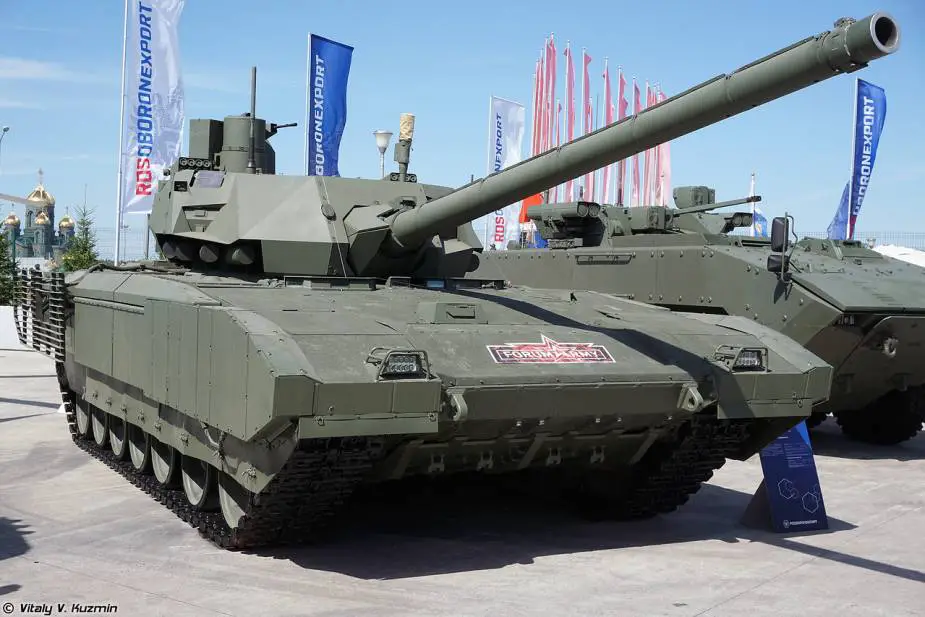A front-facing photograph showcases a prominent green tank with the barrel angled slightly upwards and to the right. The tank, which has a logo or sticker reading "Forum Army" on its front, is positioned on a concrete or paved surface. Behind it, a green armored personnel carrier is partially visible. The scene is set against a clear blue sky, with several raised banners in red, blue, and white colors. Among these banners, some display "Rosoboronexport." Additionally, a blue sign is faintly discernible in front of the tank. No people are present in the picture, which appears to be taken at a military-themed event or exhibition, possibly illustrating various military vehicles and equipment.